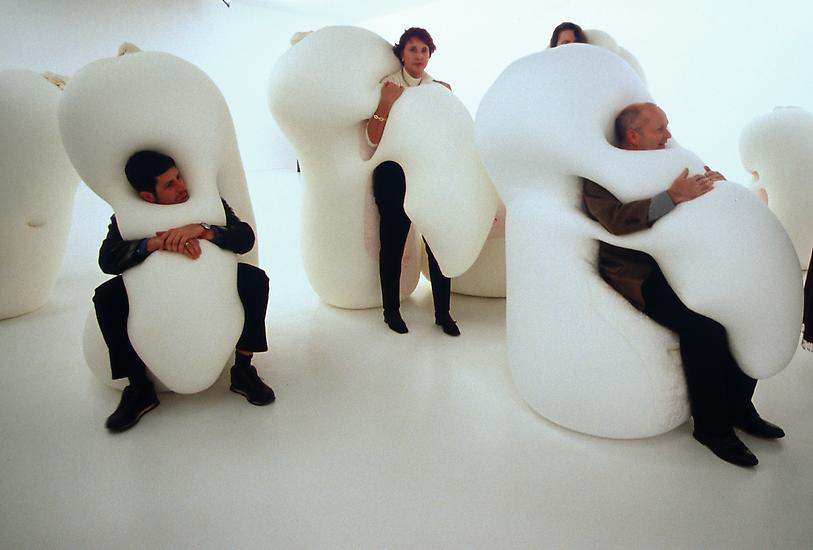The image is a landscape-oriented color photograph depicting an indoor art installation featuring interactive foam sculptures by artist Ernesto Neto. The environment has a pure white floor and an almost seamlessly blending white wall, with a light source emanating from where a wall should be in the background. The installation includes four people of Caucasian descent, each of them engaging with the large, white, bulbous foam sculptures.

On the left, a man wearing black pants, black shoes, a black jacket, and with black hair, is seated inside one of these sculptures. His arms are folded around the front of it as he looks towards the right side of the image. Next to him, a second man sits similarly on the right of the image, dressed in a black suit and gray shirt, with a receding hairline. Both men appear to be enveloped within the sculptures, which feature a unique design reminiscent of roller coaster seats or abstract teeth, fully covering their fronts and backsides.

In the center, near the top of the image, stands a woman wearing a white short-sleeved shirt and black pants. She has short dark hair and is seen standing inside one of the sculptures, which reaches from her shoulders to the floor and appears as wide as her stature. The front section of her costume-like sculpture extends down to about her knees. Another woman is partially visible to her left, showing only the top of her head.

The overall scene is set against a minimalistic backdrop enhancing the experimental and modern art style of Neto's work, showcasing how these foam sculptures envelop their participants, creating a striking visual contrast within the pristine white environment.